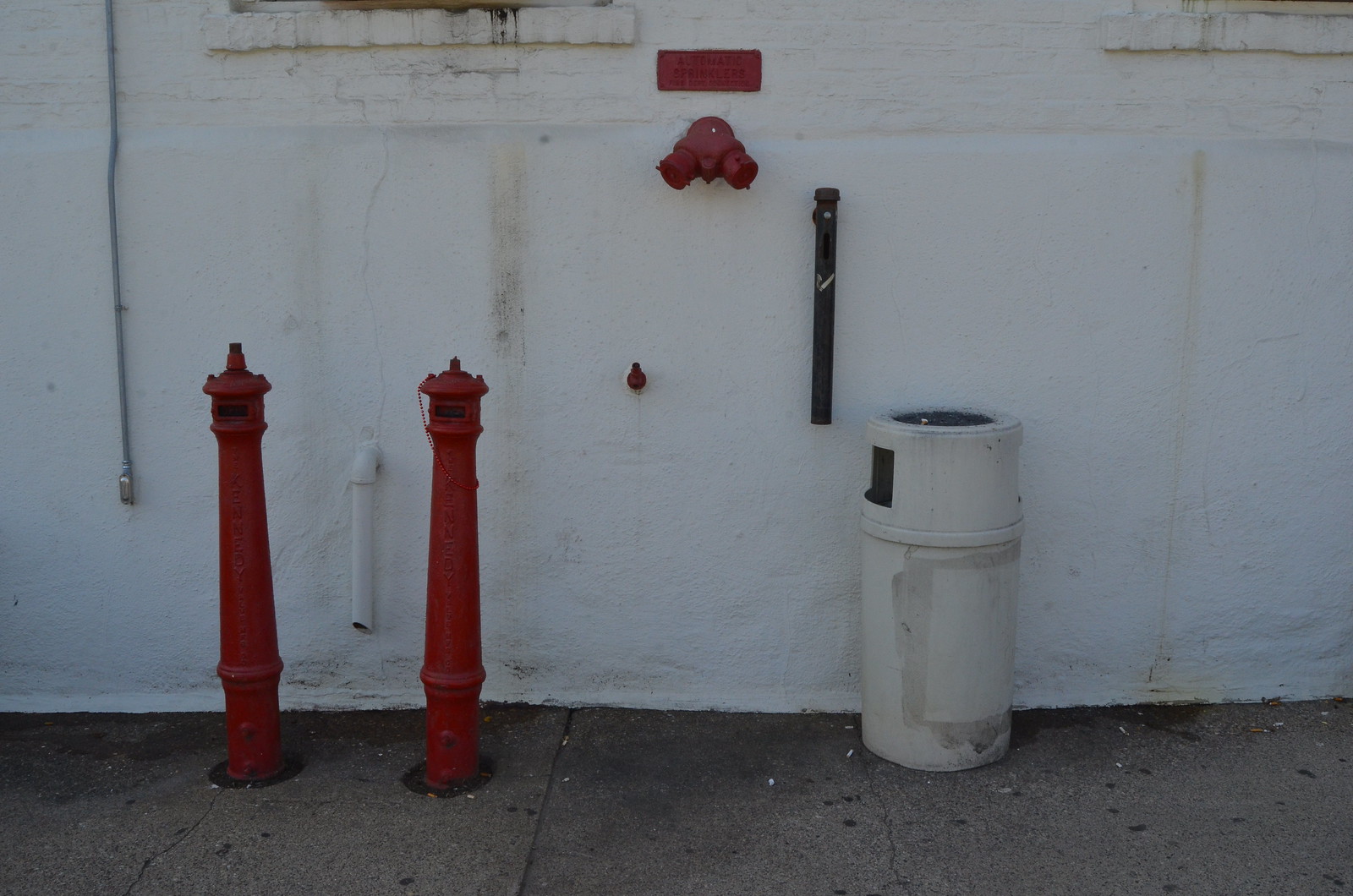The image is a horizontally long, amateur photograph capturing a slightly dim and dark scene of an outdoor sidewalk flanked by a dirty, old white-painted wall. The wall, marred with cracks, dirt, and rust stains, features various mechanical elements fixed to it. Prominently, there is a white circular trash can with a black top designed to accommodate cigarette butts, visible against the wall. The ground beneath has a dark concrete sidewalk littered with cigarette butts.

To the left of the trash can, two bright red pillars are fixed into the concrete, standing taller than the trash can and likely related to a hydro or water system. Above and to the right of these pillars is a red hose connector capped off, accompanied by a red plaque, and a red, vent-like connector. Adjacent to these features, an electrical cord runs down the wall, connected to an electrical box at the bottom. Through this jumble of components, the mechanical essence of the space is accentuated against the backdrop of the worn and weathered white wall.